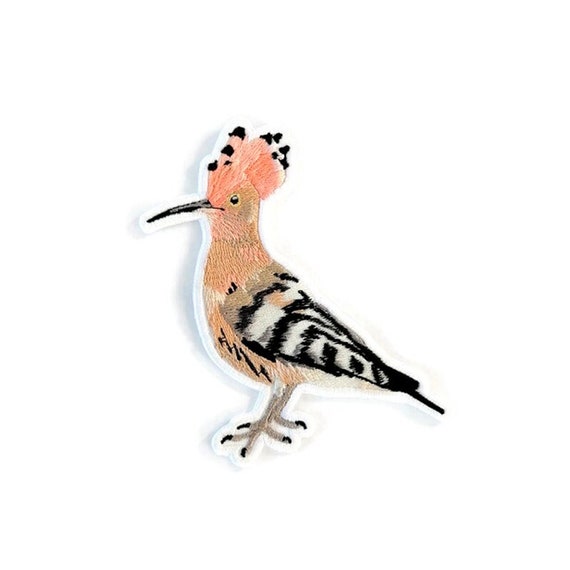This image features an intricately embroidered depiction of a small woodpecker, set against a seamless white background, suggestive of an iron-on or sew-on patch with a lightly textured, carpet-like feel. The woodpecker's feathers on top of its head are primarily light pink, accented with diagonal black circles. This detail transitions into the bird's small black eye and then to its long, slender, and pointed black beak. Moving down, the bird's neck displays subtle shades of both peach and faint pink, blending into its light brown body.

The wings of the woodpecker showcase a striking pattern: starting with dark brown feathers, it transitions into alternating horizontal stripes of black, white, black, white, and continues this pattern all the way to the pointed black tip of its tail. The bird's underbelly reveals a faint pink neck, brown body with a hint of white on the chest, and a prominent jagged black stripe. Completing the bird's physical features are its legs, which are dark gray with black nails. This attention to detail captures the unique beauty of the woodpecker in thread form.